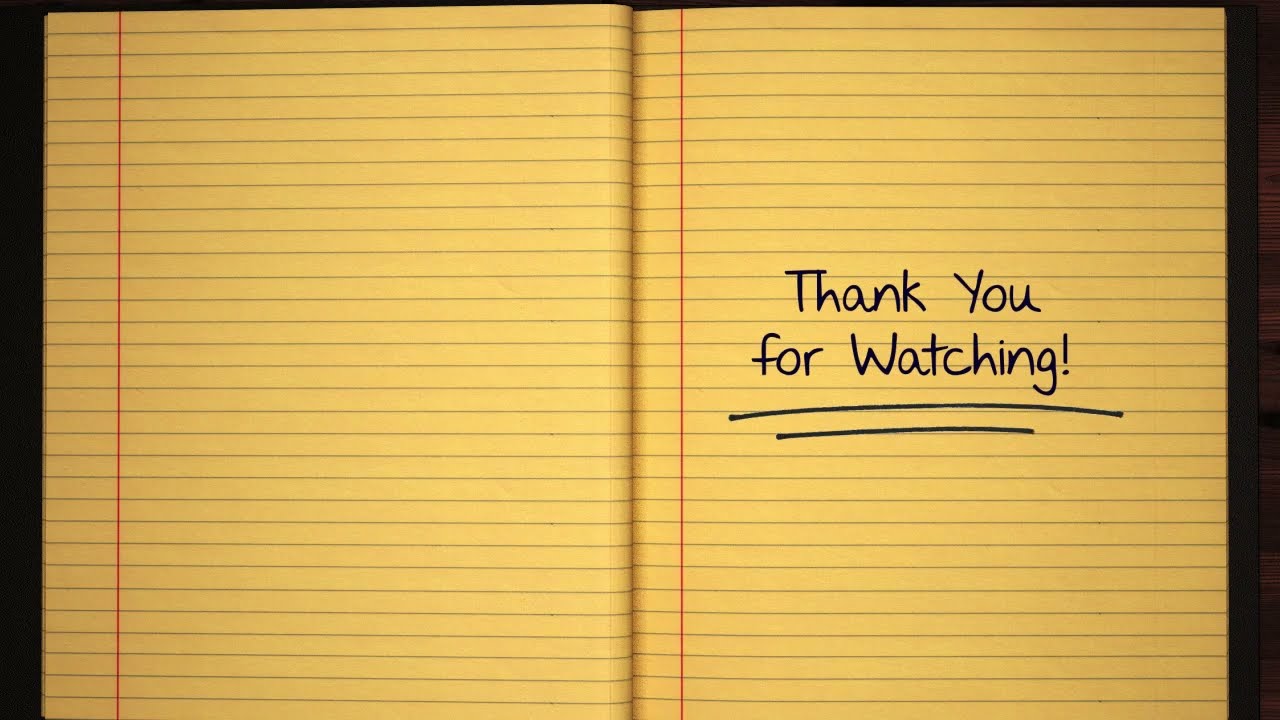The image displays an open notebook with yellow legal college-ruled paper, occupying the entire screen. The notebook is laid on a black surface, adding a subtle border on the sides. Each page is lined with blue horizontal lines and features a red margin line on the left, maintaining an organized look. The left page is entirely blank. Centered on the right page, in bold black handwriting, the text reads "Thank you for watching!" with an exclamation mark, and is underscored by two horizontal lines. The thank you message is split onto two lines, "Thank you" on the first, and "for watching" immediately below. This setup gives the impression of a digital end credit for a video or show.